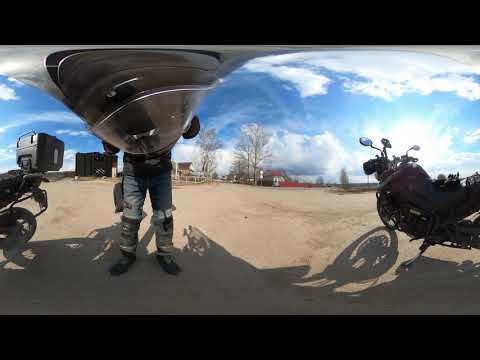This horizontally aligned, rectangular image features a daytime outdoor scene with a thick black border at both the top and bottom. The upper portion of the picture reveals a pretty blue sky, appearing slightly curved due to a 360-degree effect, with white feathery clouds at the top and puffier, slightly gray clouds lower down. The ground is a flat, sandy dirt area with a couple of barren trees and possibly some farmhouses in the background.

On the far left of the image, the back wheel of a motorcycle with a storage box is visible. The front of this motorcycle appears on the far right, leaning on its kickstand with a dark, shadowy outline cast by the sun. Near the center-left of the frame, we see a person from the waist down, dressed in ripped blue jeans, black boots, and possibly carrying a pack on the right leg, hinting at outdoor gear. The upper portion of their body is obscured by a round, gray, spaceship-like structure descending from the top of the image, possibly a distorted helmet through the 360-degree effect. There are no visible text elements, and the dominant colors include black, tan, blue, gray, and white, capturing the sandy terrain and sky's hues. This image seems to be taken in a sandy open area, similar to a parking lot or rural setting.